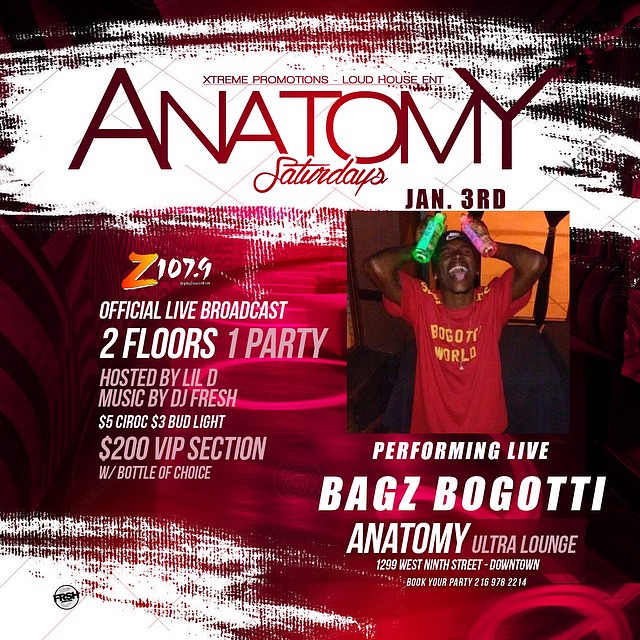The image is a vibrant and detailed poster for an event at Anatomy Ultra Lounge, located at 1299 West 9th Street, Downtown. The poster predominantly features the words “ANATOMY” in large, all-caps, reddish font, with "Saturdays" and the date "January 3rd" prominently below. The event is organized by Extreme Promotions and Loud House Ent., with an official live broadcast by Z107.9. Additional highlights include "Two Floors, One Party," hosted by Lil D, and music by DJ Fresh. Drink specials are mentioned: $5 Ciroc and $3 Bud Light, alongside a luxurious $200 VIP section offering a bottle of choice. A central image shows a smiling man in a red shirt, holding a green bottle in one hand and a reddish-pink bottle in the other. He is identified as Bags Boghoti, who will be performing live at the event. The poster's color scheme includes shades of white, black, red, pink, maroon, green, yellow, orange, and tan, giving it a festive and energetic feel. Interested guests are encouraged to book their party by calling 216-978-2214.